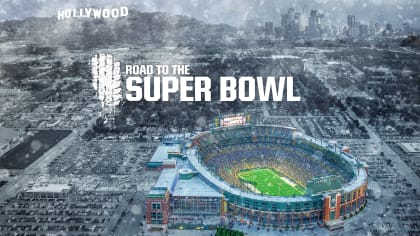The image is an aerial view of a football stadium in Los Angeles, California, depicted in a low-resolution, pixelated graphic. The stadium, vibrant with its bright green field and illuminated surroundings, stands in contrast to the gray and blurry background of the cityscape, which may depict adverse weather conditions. In the distance, the downtown Los Angeles skyline with its tall buildings is visible, adding to the urban setting. At the top left corner of the image, the iconic Hollywood sign in bold, white capital letters can be seen nestled in the mountains. Across the center of the picture, white text boldly declares, "Road to the Super Bowl," accompanied by an image of tire marks adjacent to the sign. The overall composition emphasizes the stadium and significant landmarks, creating a striking juxtaposition between the colorful centerpiece and its monochromatic surroundings.